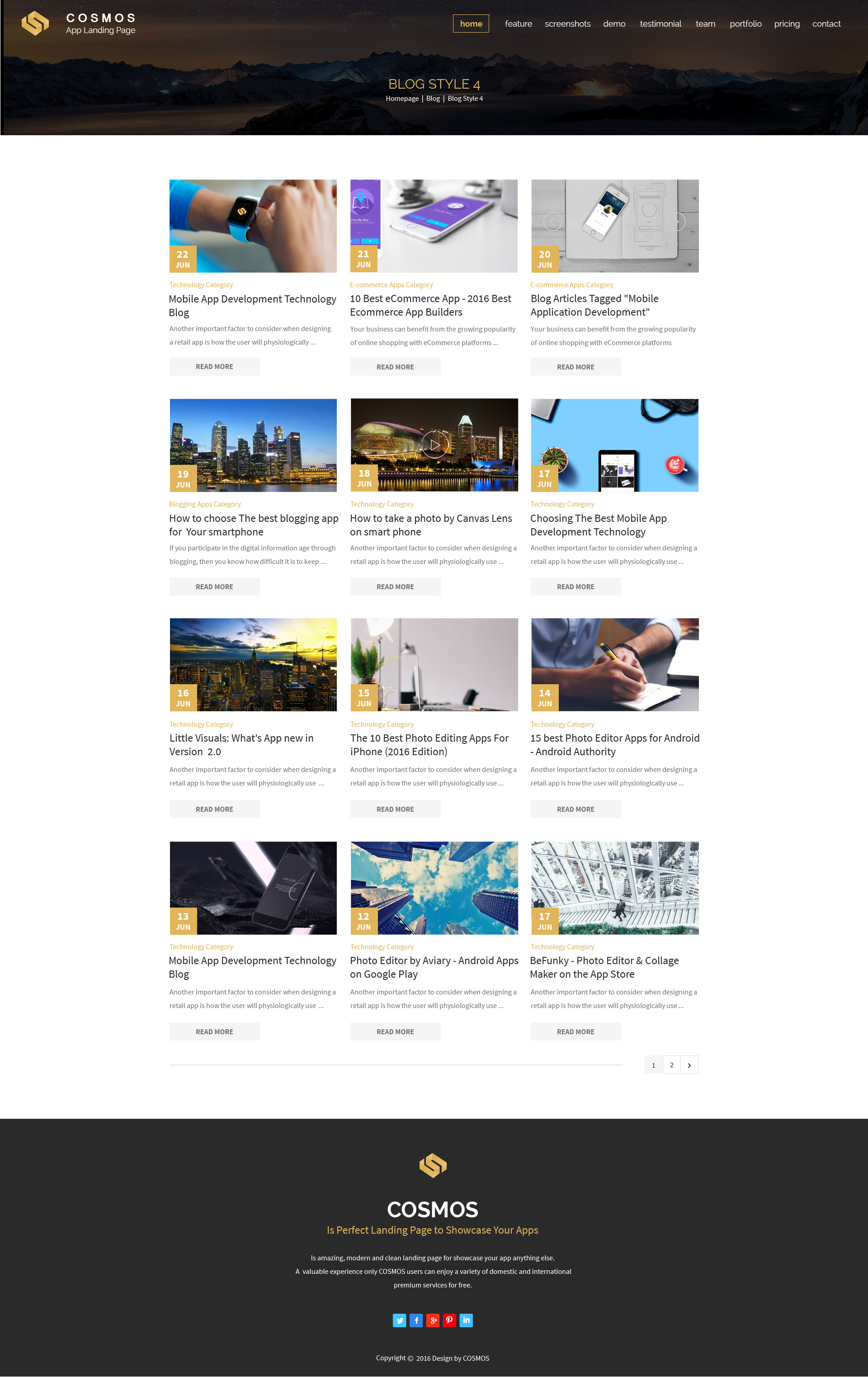In this image, a snapshot of a webpage titled "Cosmos App Landing Page" is displayed. The layout reveals a structured and organized collection of various articles, totaling twelve in number. Each article is accompanied by a date, all of which pertain to the month of June. The articles cover a range of topics related to mobile applications and technology.

Some notable article titles featured include:
- "Mobile App Development Technology Blog"
- "The 10 Best Photo Editing Apps for iPhone, 2016 Edition"
- "Photo Editor by Avery, Android Apps on Google Play"
- "BeFunky, Photo Editor and Collage Maker on the App Store"

At the very bottom of the page, a prominent banner is displayed with the text: "Cosmos is the perfect landing page to showcase your apps." This suggests that the webpage serves as a platform for users to both upload and discover mobile apps, potentially functioning as a news website focused on app-related content.